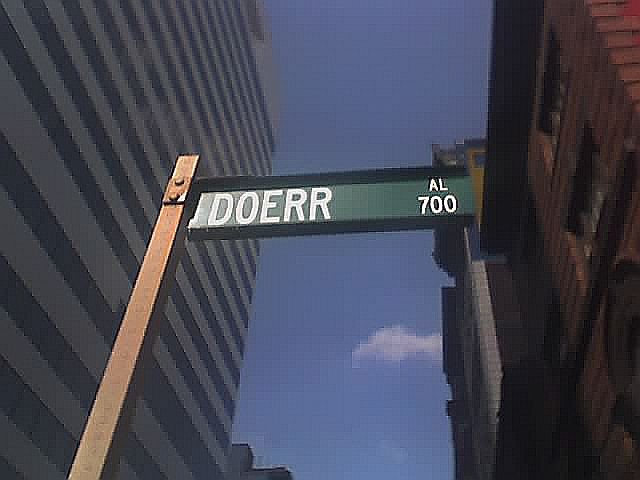The photograph captures an urban scene featuring a green street sign with the text "Doerr AL700" in bold white font. The sign is mounted on a rusted, yellow-bronze square pole. In the background, the city's skyline is visible; on the left, there is a gray building with blackish-blue horizontal stripes on its windows, while on the right, a red brick building stands adjacent to another gray structure with a yellowish upper section. The viewpoint of the image is from below, gazing upwards towards the sign and the buildings. Above, a clear blue sky with a single white cloud completes the composition, giving the scene an almost artistic quality with modern, straight brushstrokes.